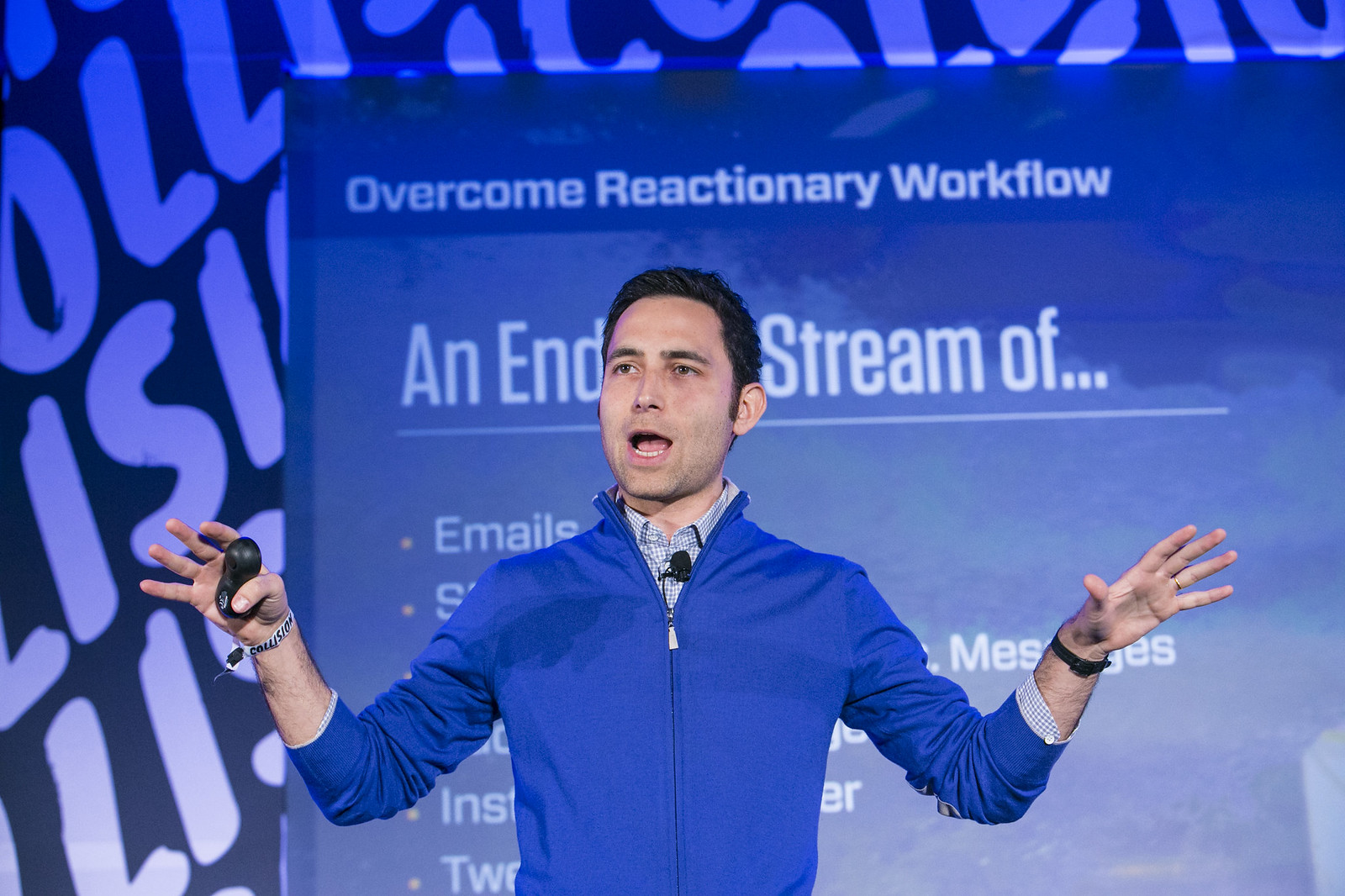In the photograph, we see a male presenter of Caucasian descent with short dark brown hair, wearing a blue zip-up jacket over a striped button-up collared shirt, to which a microphone is attached. His left hand holds a black round presentation clicker, and a wristband labeled “collision” is visible. He is standing in front of a large blue projection screen, speaking with his head turned slightly to the left and his mouth open. The screen behind him features white bold text including the phrases “overcome reactionary workflow” and “end stream of,” along with a bulleted list starting with “emails.” The rest of the text is partially obscured by the presenter. The background surrounding the presenter and the screen is also blue, with large white letters, partially spelling out “O-L-L-I-S.”